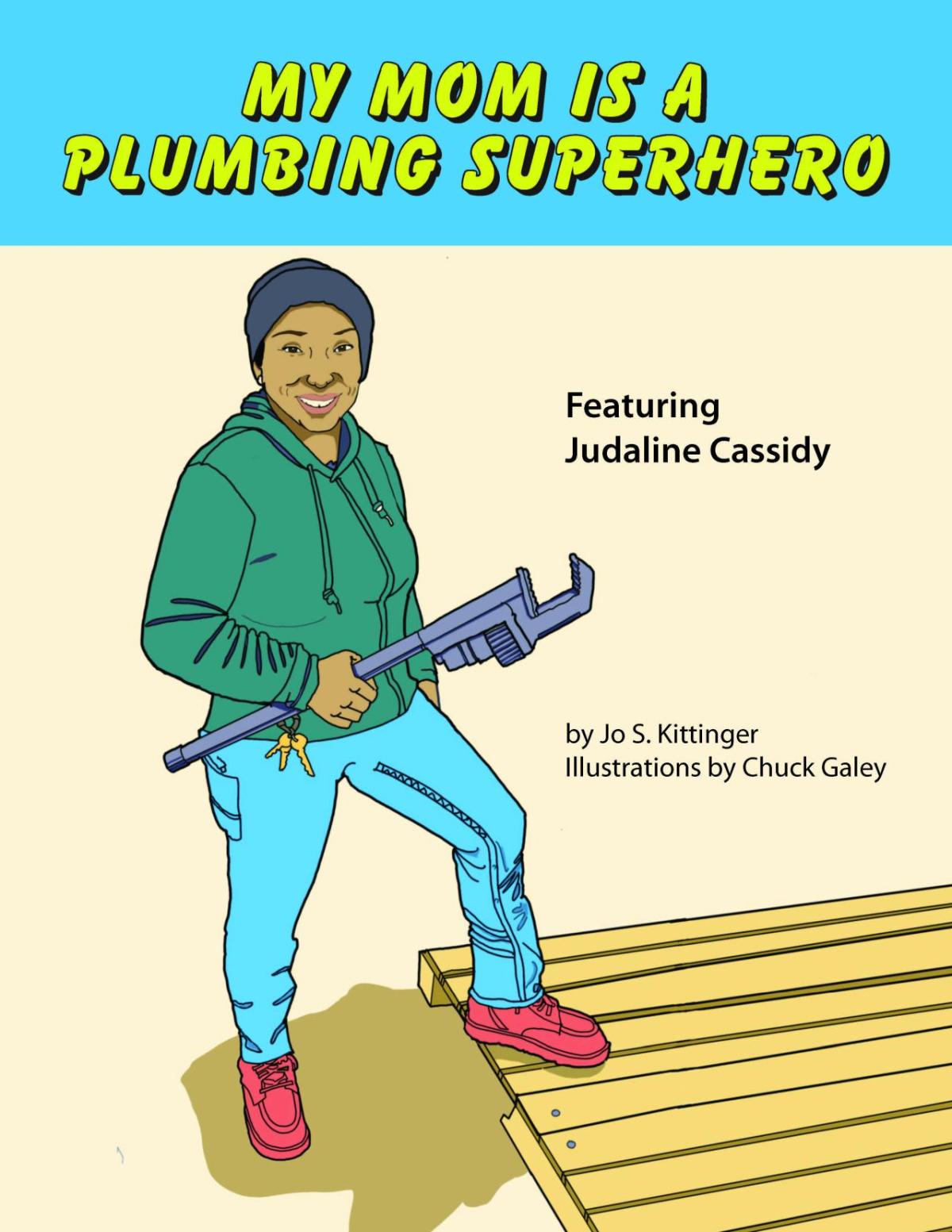This is the cover of a children's book titled "My Mom is a Plumbing Superhero". The title is displayed at the very top in bright green comic-like font on a baby blue background. Below the title, the text reads “featuring Judaline Cassidy” by Joe S. Kittinger with illustrations by Chuck Gatley, all in black letters. The background of the illustration is a tan beige color. Central to the image is a cartoon drawing of an African-American woman, smiling happily and looking directly at the viewer. She is wearing a black or navy blue beanie, a green zip-up hoodie with visible hoodie strings, light blue pants, and red shoes. She holds a large plumber's wrench in her right hand and has some gold keys dangling from her pocket. One of her feet is firmly placed on a wooden slat or pallet as she stands confidently against the plain background.